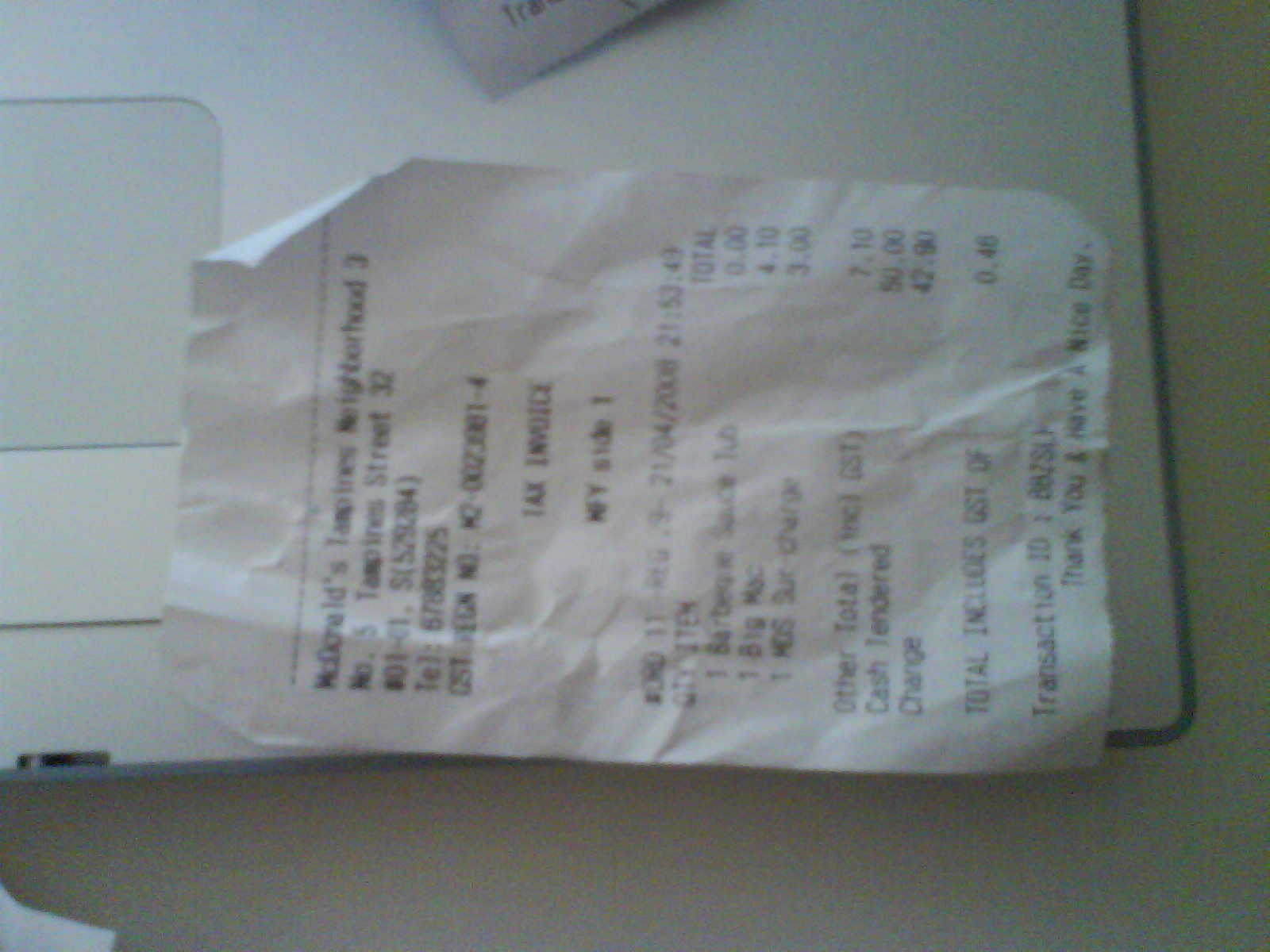A close-up, angled view captures a tiny McDonald's receipt resting horizontally on the bottom right corner of a laptop keyboard. The trackpad of the laptop is visible in the upper right section of the image, while a portion of a white table is discernible at the bottom. The receipt's top part, which lists McDonald's, is oriented towards the left, and the bottom part of the receipt, containing the total, faces right. Although some details on the receipt are blurry, it's clear that the total expenditure was $7.10. The customer paid with a $50 bill and received $42.90 in change.